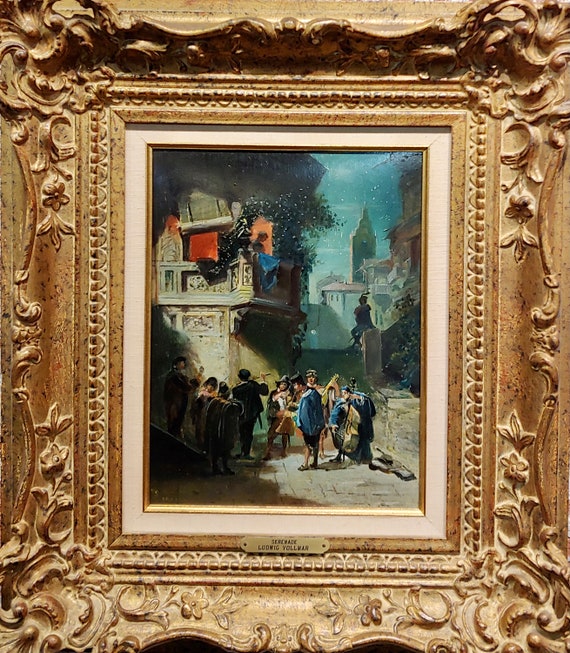The image is a detailed and vibrant painting set within an extremely ornate, hand-carved frame that takes up significant space and features intricate swirls, flowers, and leaves on the corners and sides. The frame, with a dull goldish-brown hue, boasts a small gold nameplate at the bottom that reads "Serenade Locking Vollmer." This luxurious frame surrounds a white matte border that leads into the main painted scene. The painting depicts a vintage, outdoor moment where several suitors with various musical instruments, such as guitars, flutes, and string instruments, stand beneath an old, orange-colored, palace-like building. Some of their carrying cases are strewn on the ground. One musician plays bravely while another, seemingly too shy or fearful to speak, stands with his head down. Above them, on a balcony, a young woman looks down at the scene, capturing the essence of a serenade from a bygone era.